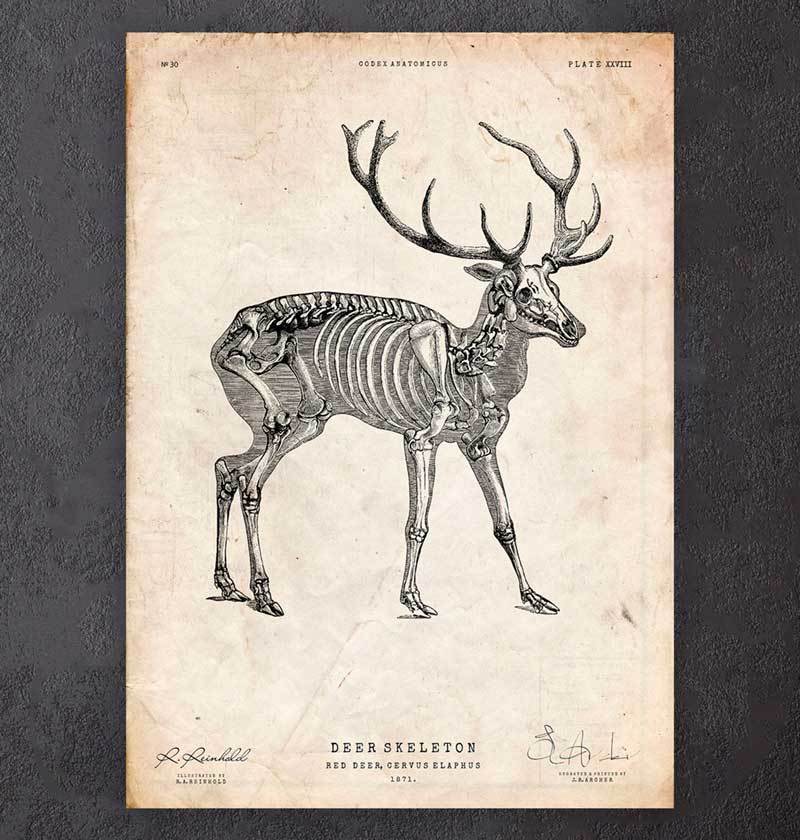The image depicts a vintage, biology textbook-style illustration of a red deer (Cervus elaphus), emphasizing the skeletal structure overlaid on the deer's outline. The deer boasts a large set of antlers with at least an 11-point rack, and beneath the central figure, the caption reads: "Deer Skeleton, Red Deer, *Cervus elaphus*." The illustration itself is set against an aged, wrinkled, and slightly tattered beige canvas, showing signs of wear particularly at the top edge. Unreadable text is located in the top center, possibly including the title and "Plate XXVIII" in the upper right corner. Two illegible signatures appear in the bottom left and right corners, likely belonging to the artists. The overall aesthetic of the image exudes an old-school, vintage charm.